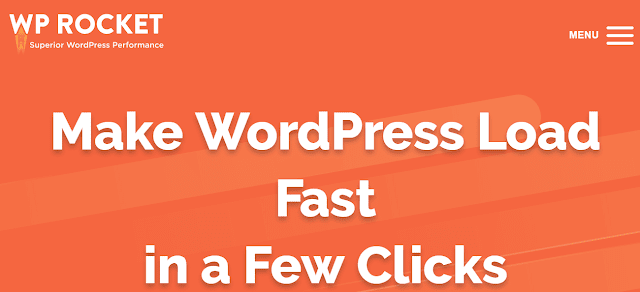The image appears to be a cropped section of a web page, specifically focusing on the header graphic with an orange-hued background. The background color is not uniform; it features a subtle pattern of diagonal rectangles where the orange is slightly lighter, giving it a nuanced texture.

In the upper left-hand corner, the company name and logo are prominently displayed in white, capital letters, reading "WP ROCKET." Beneath the "W" of "WP ROCKET," there is an arrow symbol, subtly lighter in orange compared to the background, which adds to the visual branding.

Below the logo, the tagline "Superior WordPress Performance" is written in white with initial capital letters. Centered in the middle of the header is a large headline in white font, declaring, "Make WordPress Load Fast in a Few Clicks."

On the upper right-hand corner, the word "MENU" is displayed in white capital letters, followed by three horizontal white lines signifying a menu icon. This overall design conveys a clean, professional, and performance-oriented aesthetic.